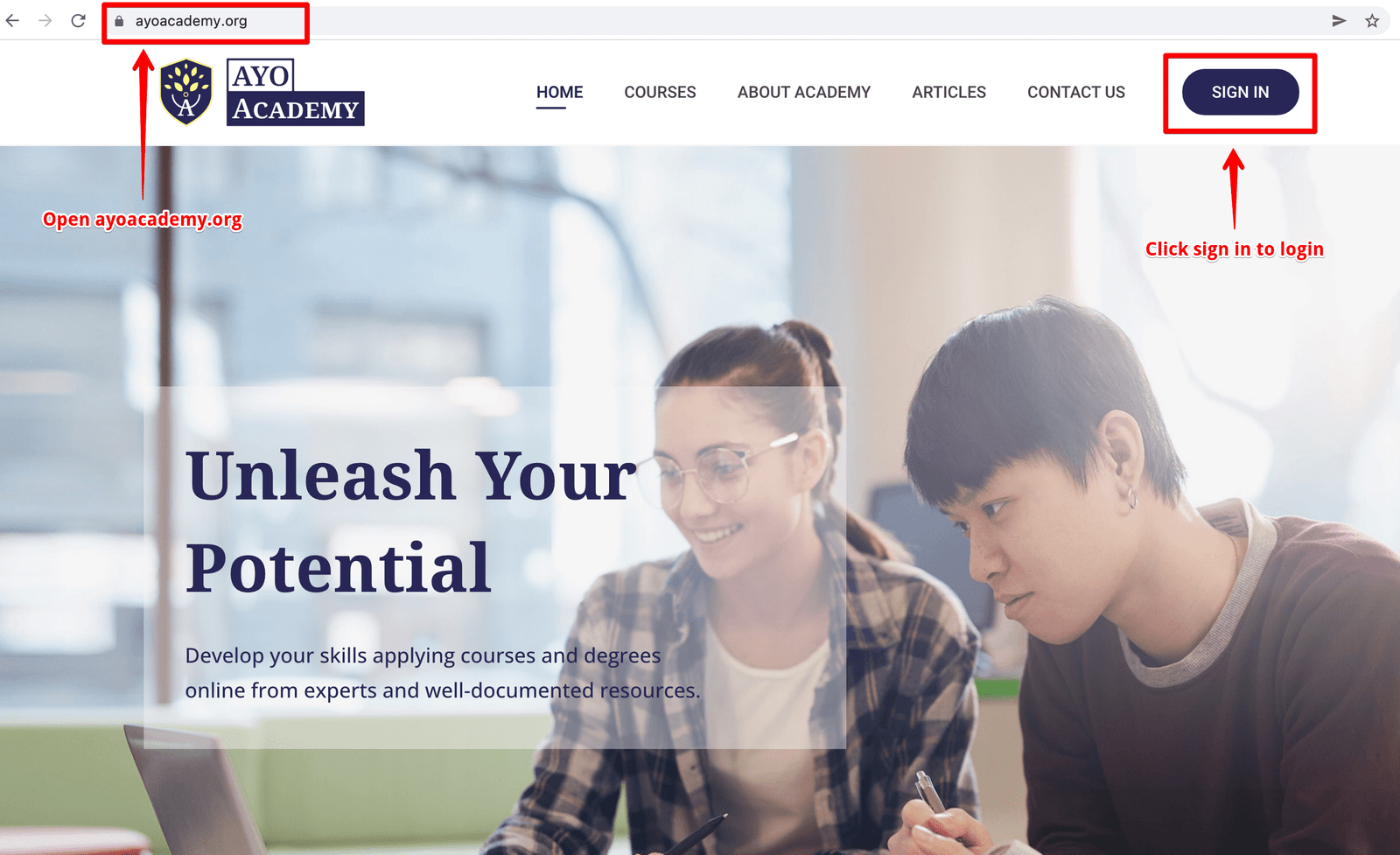The screenshot features a detailed interface of the website aoacademy.org. At the very top, the URL bar displays aoacademy.org, highlighted by a dark red rectangular border. A thick, red arrow points towards the URL bar, narrowing down to a text bubble outlined in white, which reads "Open aoacademy.org."

Beneath the URL bar, on the left side, there is a logo composed of a dark blue shield adorned with yellow tree leaves at the top. Inside the shield, a white letter 'A' is positioned at the bottom, accompanied by two white curved lines.

To the right of the logo, the text “AYO” is prominently displayed in all capital letters, resembling a Times New Roman font. It is set against a white background with a dark blue border. Directly below, within a dark blue rectangular icon, the word “Academy” is written in the same font and capitalized in white.

Further to the right, a navigation menu is present. The menu options include: "Home" (underlined, indicating it is the current selection), "Courses," "About Academy," "Articles," and "Contact Us." On the far right, an oval-shaped button with a dark blue background stands out, inscribed with “Sign In” in white capital letters. This button is also highlighted by a dark red rectangular border, with a similarly constructed red arrow pointing towards it. The accompanying text bubble reads "Click Sign In to Log In."

Towards the bottom right of the webpage, an image features a man and a young girl intently looking at a computer screen. The girl, who has a braided hairstyle, glasses, a plaid shirt, and a white undershirt, is smiling. Overlaying this image is a semi-transparent dark blue text box that states: "Unleash Your Potential." Below this headline, smaller blue lettering reads: "Develop Your Skills Applying Courses and Degrees Online from Experts and Well-Known Resources."